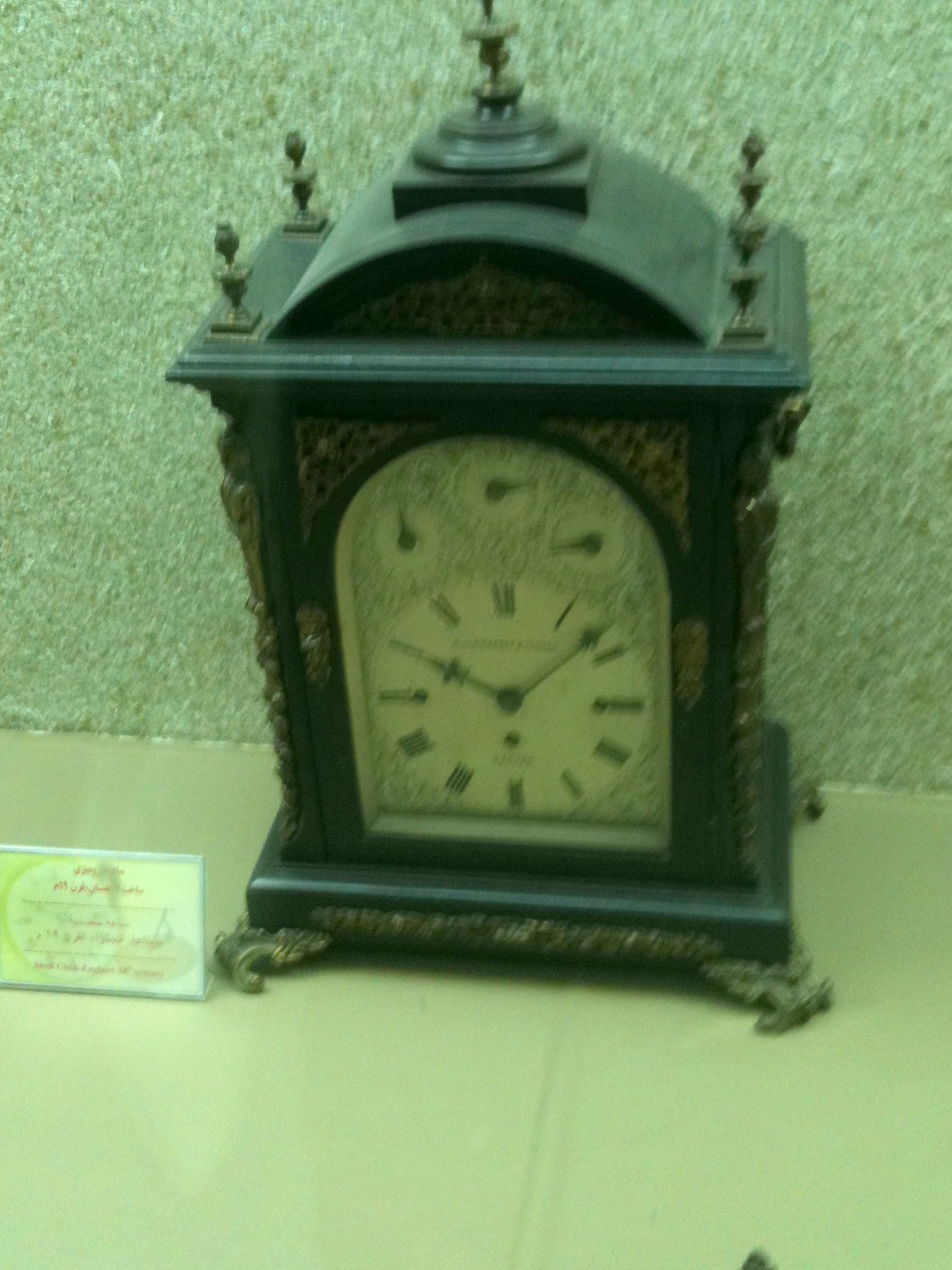This photograph features an intricate, antique mantel clock, captured from an above-angle. The clock itself is primarily a dark wood with gold claw-style feet and ornate gold decorations adorning its sides and bottom. It has an arched top crowned with a prominent finial, and each corner underneath the arch is marked by smaller finials. The clock's face, set against an off-white background, displays Roman numerals with black hour and minute hands indicating roughly seven minutes past ten. The face also features a decorative swirled design.

The setting of the photograph appears to have a yellowish tinge, possibly due to the lighting or a filter, giving both the clock and surrounding area a light greenish hue. The clock is placed on a surface that seems to be beige or light green, with a small card featuring what appears to be Arabic script in red against a yellow gradient background positioned to its left.

The background wall is mottled in dark and light shades, contributing to the filtered appearance of the image. The photograph emits a slightly vintage ambiance, further enriched by the clock's embellished features and the soft lighting that casts a gentle glow over the entire composition.